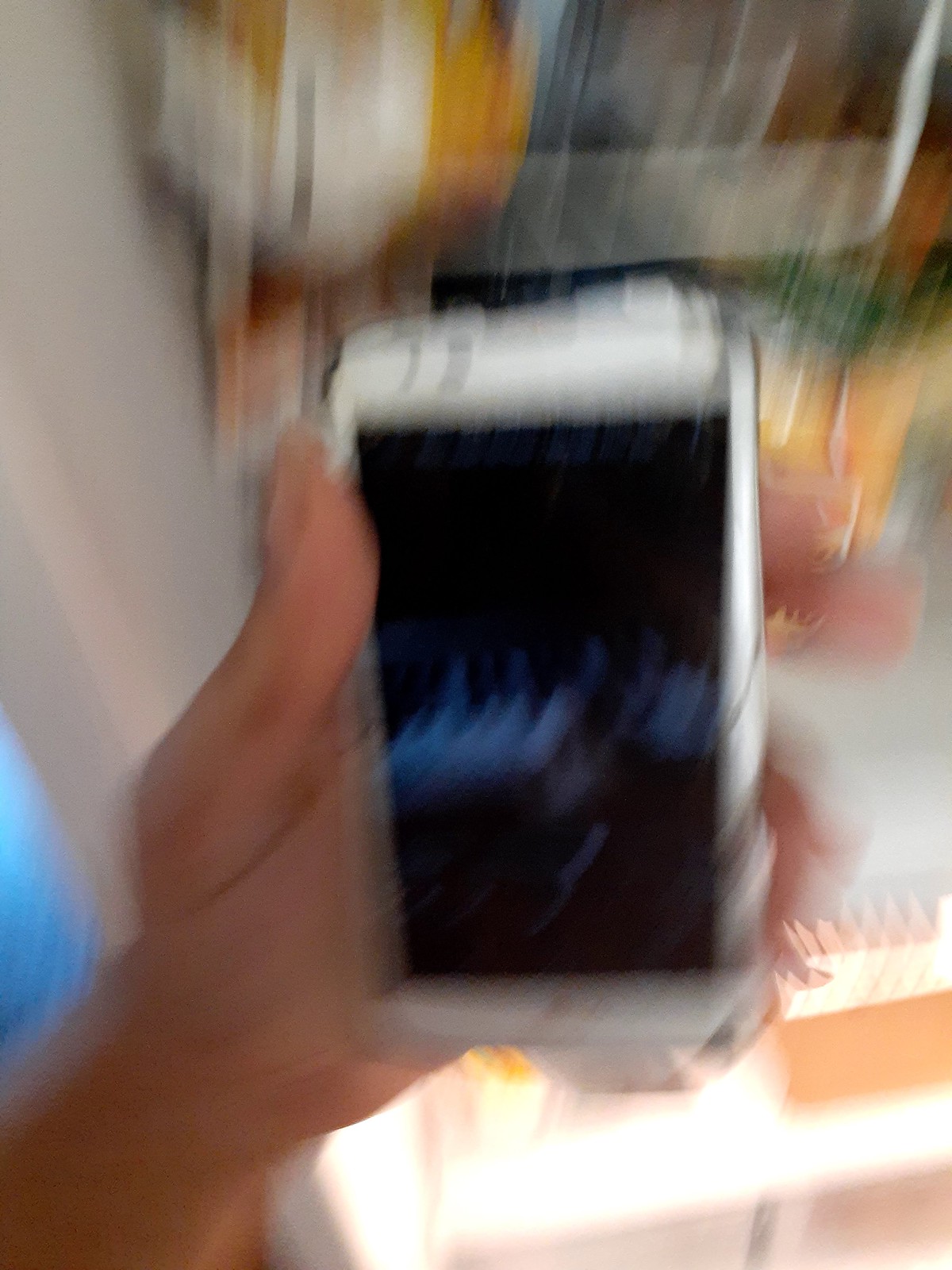This rectangular, portrait-oriented image is notably blurry, making detailed identification challenging. At the forefront, a hand makes an appearance, grasping what seems to be an older model of an iPhone. The device features a black frame interspersed with white sections, indicating likely wear and tear, and its screen is visible but appears damaged or malfunctioning. The background is a vague amalgamation of lights and indistinct objects due to the blur, adding to the image's enigmatic quality. A particularly bright light source emanates from the bottom, casting a glowing effect upward. On the left side of the image, a blue patch is visible, possibly the sleeve of a shirt worn by the person holding the phone.